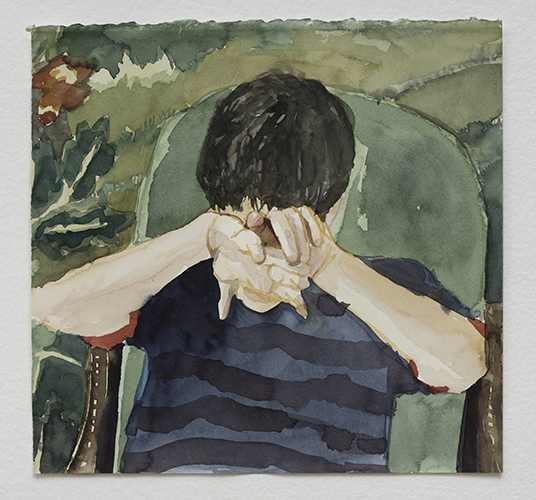This watercolor painting depicts a young boy with short black hair, sitting in a green chair. He appears to be upset, burying his face in his hands, with his elbows bent and fingers interwoven in various positions. His attire includes a blue shirt with darker blue, almost navy stripes, complemented by red sleeves. The boy's posture and his obscured face suggest an emotional moment, as though he might be crying. In the background, there is a blend of greenery with leaves and a striking red flower. The watercolor style is evident in the soft blending and drips on his skin and shirt, giving the image a slightly unfinished, blurred effect. Additionally, the painting features a subtle gray framing around its edges.